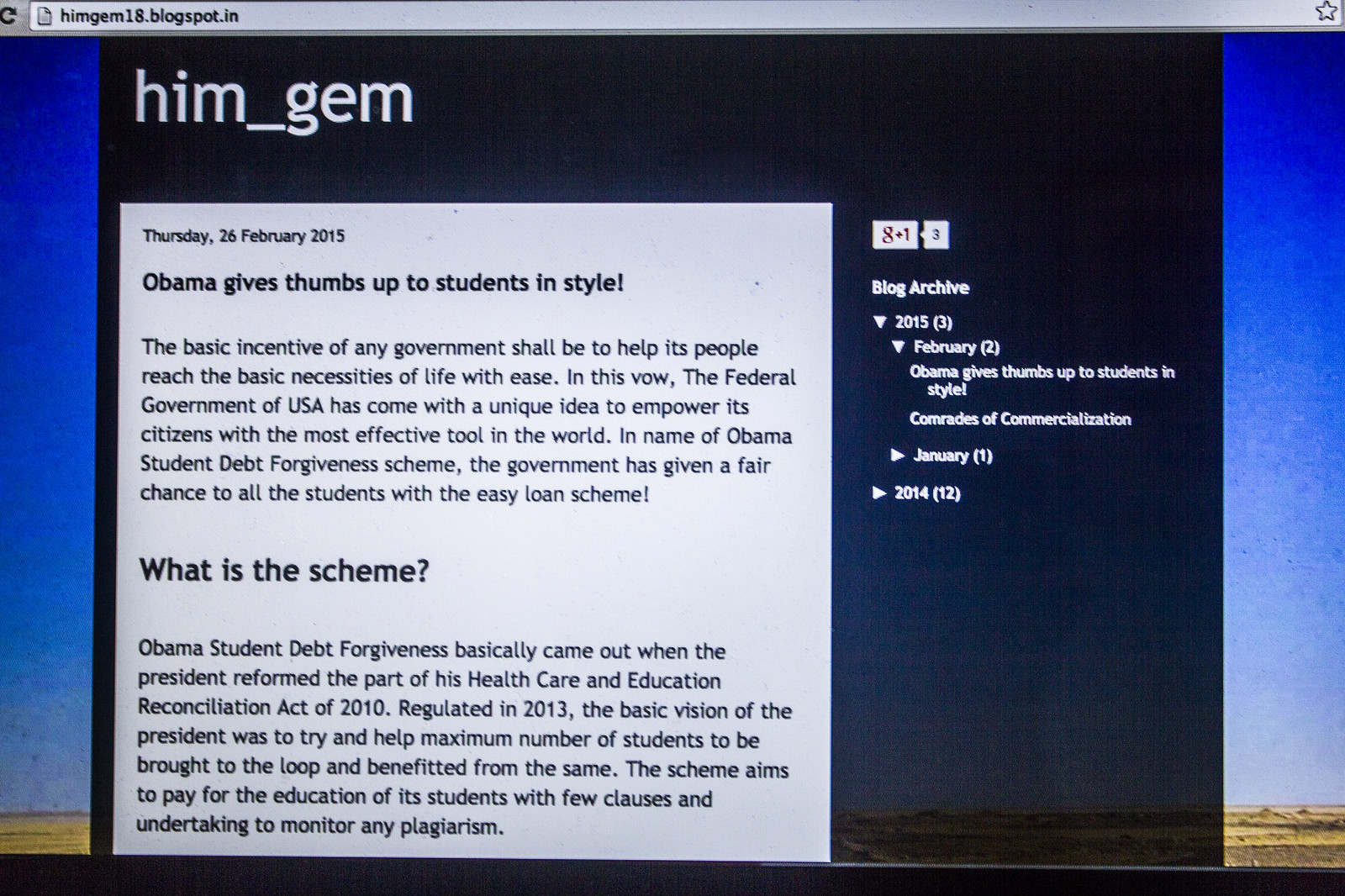This image captures a screenshot of a blog website with the URL himgem18.blogspot.in. The blog, titled "Hem_Gem," features a post dated Thursday, 26 February 2015, with the headline "Obama Gives Thumbs Up to Students in Style." The overall layout includes a white background for the main content area, bordered by dark blue on the right and left, with white text on the blue borders. On the right side, there is a navigation bar labeled "Blog Archive," listing posts from 2014 and 2015. The main content discusses the Obama Student Debt Forgiveness Act of 2010, regulated in 2013, which aims to help students manage educational expenses under the Healthcare and Education Reconciliation Act. The scheme is described as a government initiative to ease the basic necessities of life by providing an easy loan scheme for students.